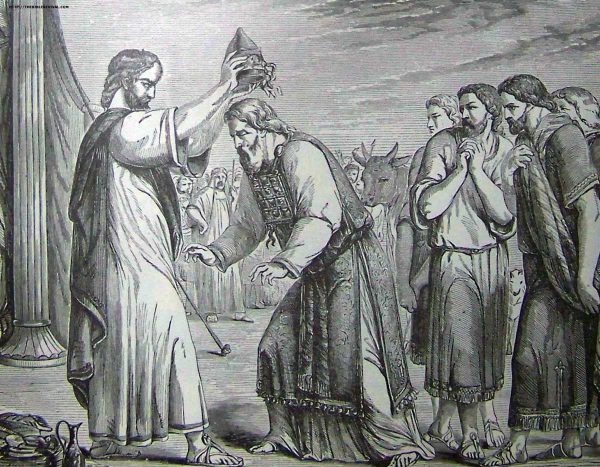The image is a detailed black and white etching depicting a significant ceremonial scene. At the center, a man in a long white robe layered with a darker robe stands with a solemn expression, placing a crown on a kneeling individual's head, suggesting the crowning of a new leader or dignitary. To the right of the kneeling man, a group of onlookers stands, their expressions ranging from displeased to judgmental, hinting at a possible controversy or mixed feelings about the event. In the background, to the left of the man performing the crowning, a single ornate pillar with multiple vertical lines flares out. Further back, behind the crowd, the rear of an oxen is visible. The sky is artistically rendered with hatching lines, creating a darker appearance without obscuring the scene, and it remains ambiguous if there are clouds present. The entire composition is in grayscale, providing a timeless and solemn atmosphere to the moment captured.